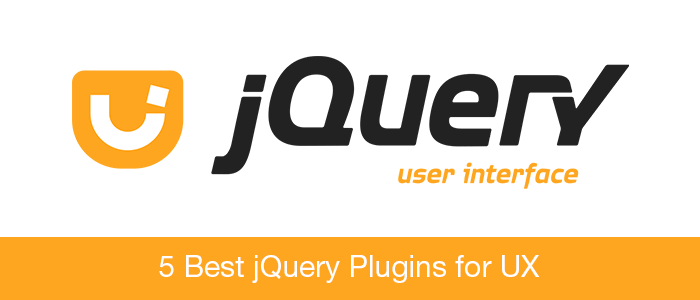The image is a rectangular graphic, three times as wide as it is tall, primarily featuring a white background for the top 75% of its area. Dominating this section is a notable logo and text design. On the left side, occupying the area starting roughly 10% from the left edge and stretching to about one-third of the width, is an orange, filled U-shape that transitions into a square form at the top. Inside this orange shape lies a white U-shape, which diverges at the upper right corner, giving the impression of breaking off towards the right - forming a distinctive logo.

Adjacent to this logo, on the right side, is the word "JQUERY" in large, bold, black letters occupying about a third of the image's height, with the 'J' in a larger font followed by uppercase "QUERY." Below and slightly to the right of this, in smaller orange text, are the words "user interface."

The bottom 25% of the image features a solid orange background block. Centered within this block, in large, white uppercase text, it reads: "5 Best jQuery Plugins for UX," with notable capitalization on "Best," "Query," "Plugins," and "UX."